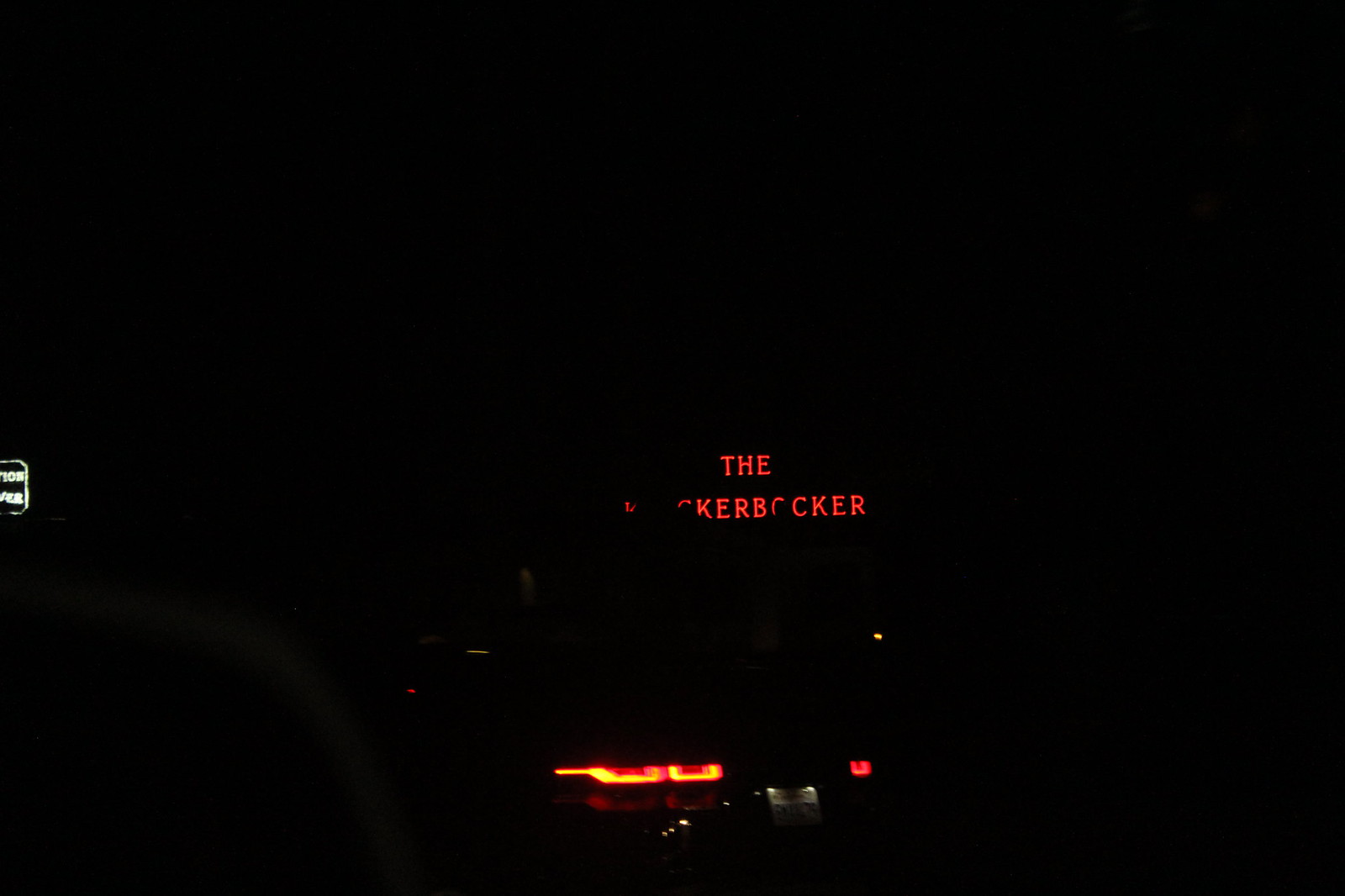The image depicts a mostly black frame with a central focus on a neon sign featuring bright red letters. At the top, the sign reads "THE," followed by three blurred characters due to a black obstruction, then illuminates the fragmented word "KERBOCKER" in red neon light. Further below, the image appears faintly lit by a set of orangish-red lights, likely taillights from a vehicle. To the far left, there's the barely discernible outline of another sign in black with white lettering and a white outline. The backdrop is entirely pitch black, suggesting it might be an exterior nighttime scene, potentially viewed from within a vehicle, hinted at by the dim shape of a possible steering wheel in the bottom left.